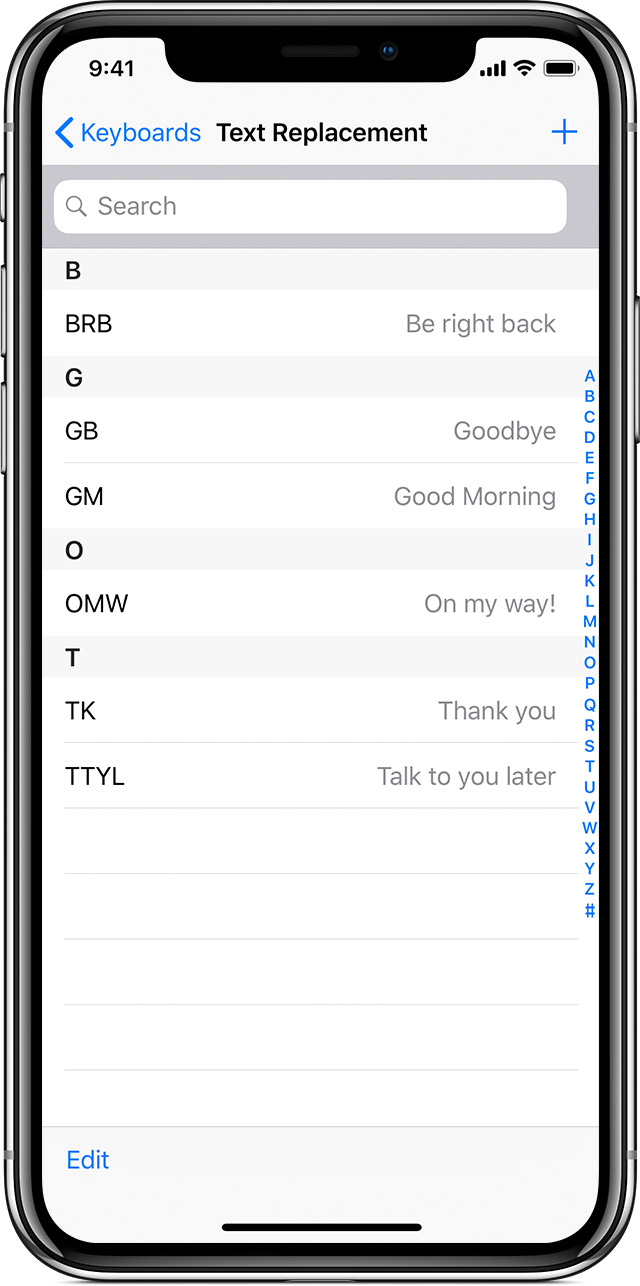The image displays the screen of a mobile device, likely an iPhone, showcasing the "Text Replacement" settings. At the top, the navigation option "Keywords" is highlighted in blue, indicating that it serves as a link to return to the previous screen. The primary section of the screen features a search bar, inviting users to input search terms. Below the search bar is a list of text replacement entries where abbreviations are paired with their corresponding phrases for automatic substitution during typing. The entries include: "BRB" for "Be Right Back," "GM" for "Good Morning," "TK" for "Thank You," "TTYL" for "Talk To You Later," "GB" for "Goodbye," and "OMW" for "On My Way." This setup allows users to create shortcuts for frequently used phrases, enhancing typing efficiency.